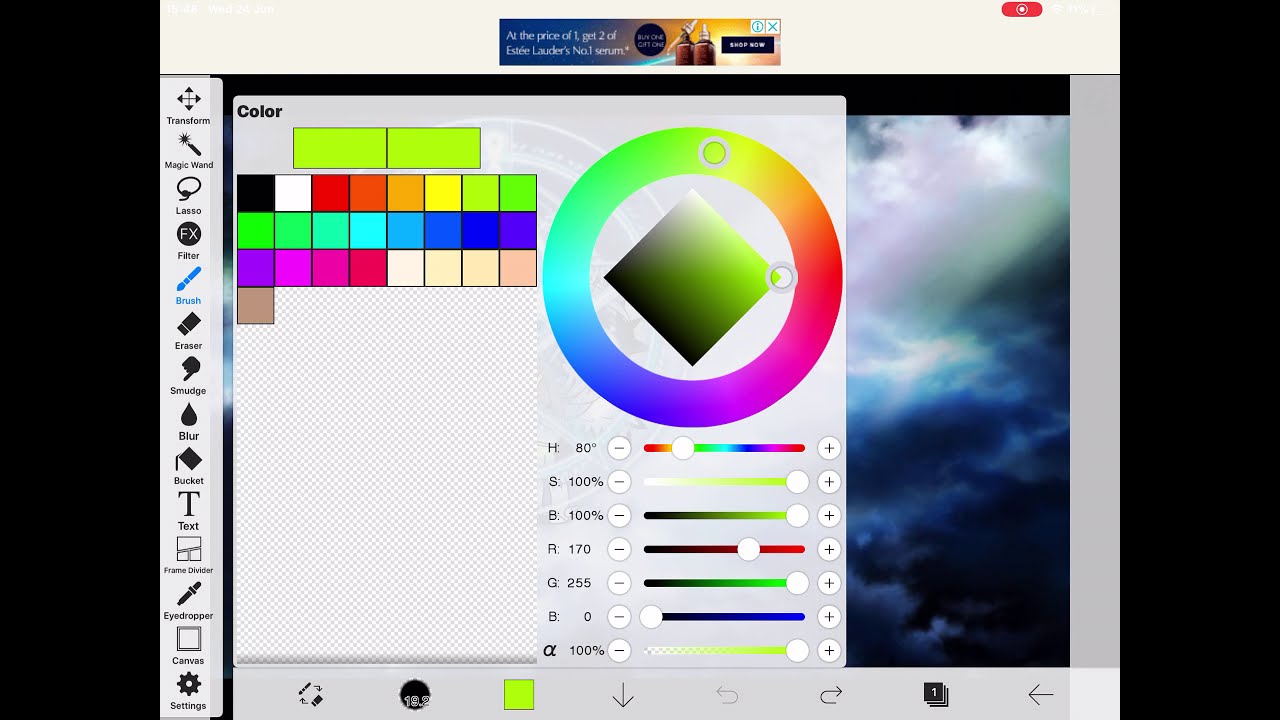The image depicts the user interface of a web-based picture editing software, with both left and right vertical black bars occupying around 10-15% of the screen. On the left bar, a variety of tool icons are visible, including options like transform, magic wand, lasso, brush, eraser, smudge, blur, bucket, text, eyedropper, and settings. There is also an advertised banner at the top, indicating a web environment. The center of the screen showcases a colorful, dark-to-light gradient diamond within a rainbow-colored circle. Below this diamond are lines of text interspersed with white circles, rainbow-colored lines, and black specks of writing. Additionally, on the left side of the central design, there are two lime green rectangles and a grid of around 30 small squares in a 3x10 arrangement, featuring random colors like black, white, red, orange, yellow, and green. On the right side, a color palette with a color wheel and customizable sliders is visible. In the background, the image being edited shows a sky with a blue, cloudy appearance.